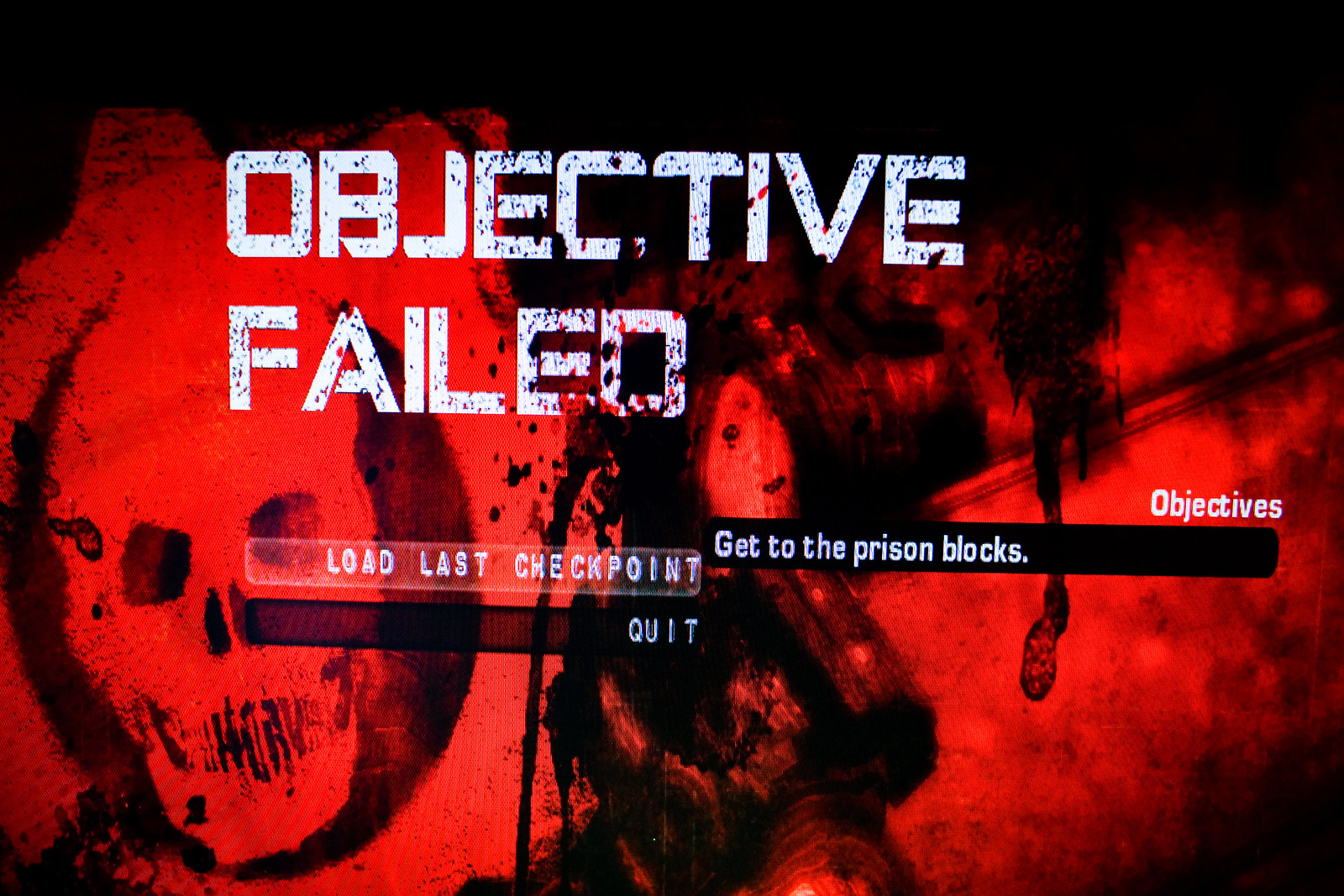The rectangular image features a predominantly black and red background adorned with jaggedly-toothed skull shapes, creating a dark, ominous visual. At the center, there is a distorted, potentially female figure with long hair, seemingly dressed in a black or dark garment. The background imagery and the figure appear to be dripping with black and red splatters, enhancing the eerie atmosphere.

Across the top in bold, white letters is the phrase "OBJECTIVE FAILED," accompanied by blood splatter, indicative of a failure or death screen in a video game, likely "Gears of War." Below this, the text "OBJECTIVES" appears in white, followed by "get to the prison blocks" on a black band. Further below, the options "load last checkpoint" and "quit" are listed, with "load last checkpoint" appearing in a transparent white highlight.

On the left-hand side, the recognizable Gears of War logo is prominently displayed, adding to the game's thematic elements. The right-hand side of the image contains blurred, indistinct visuals, potentially including more blood drips, contributing to the unsettling design. The overall color scheme of red, black, and white text effectively conveys the sense of danger and urgency typical of the game's aesthetic.